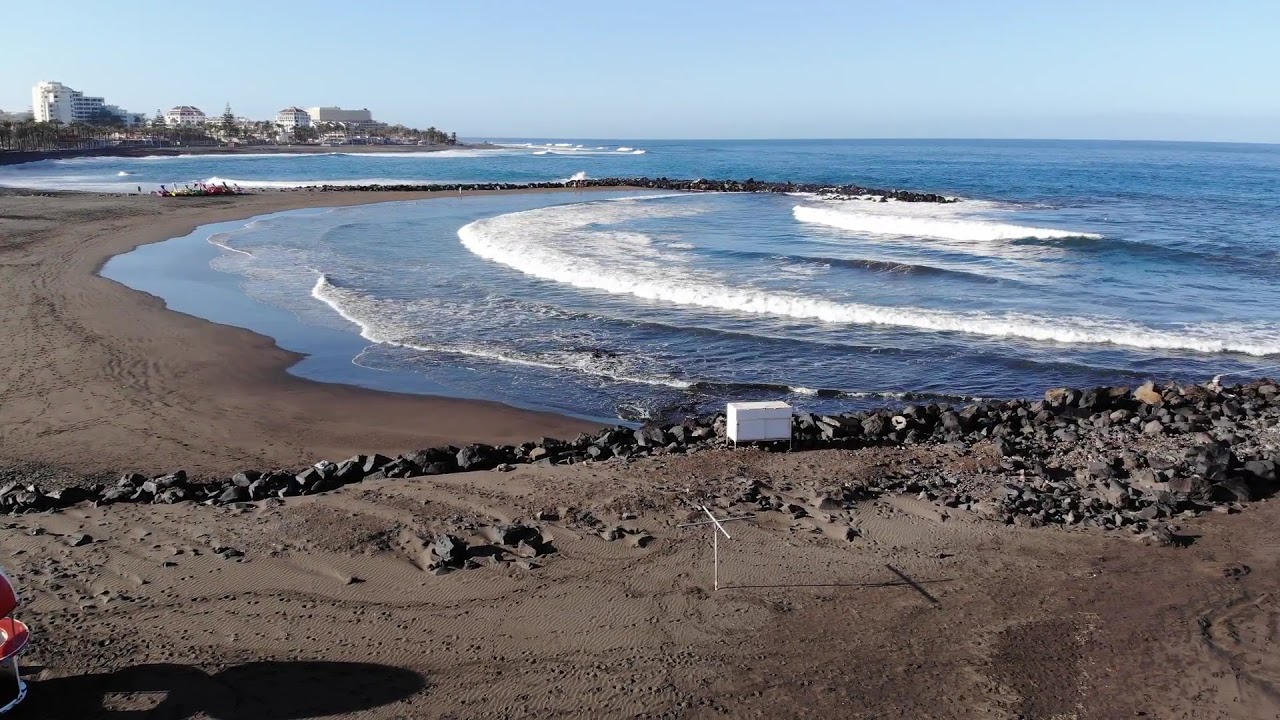This photograph captures a vivid seascape with the right side dominated by the sprawling blue ocean, while the left side features a beach with dark, brown, and gravelly sand interspersed with numerous stones. The beach extends towards the middle of the sea in an elongated promontory. The ocean itself possesses varying hues of blue, with white-tipped waves created by the tumult of the sea. In the foreground, scattered near the shore, are a few indistinct figures, suggesting human presence, and a red object resembling a chair at the very left corner, along with a white, rectangle-like structure near the center bottom right.

The top left of the photograph showcases some tall buildings, potentially condos or hotels, stretching hazily up into a light blue, clear sky. These buildings are accompanied by a few scattered trees, and their placement suggests a slight dip in the land as it meets the shore. The entire scene is set in the daytime, reflecting a bright and crisp atmosphere.